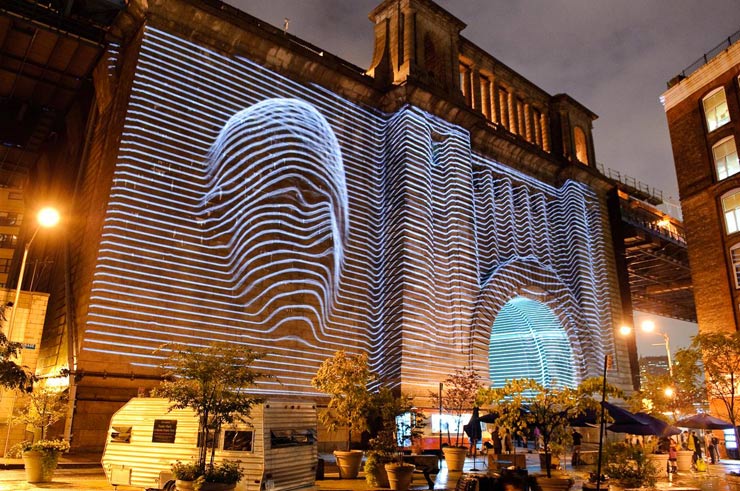The photograph captures a dynamic city scene at night. Dominating the image is an old brick building with Greco-Roman architectural elements, featuring a striking overpass with classic columns. A highly detailed and captivating work of art is displayed on the side of this structure, possibly achieved through projection or light tubes. The artwork consists of horizontal light bars that create the illusion of a giant face emerging from the building, extending into the tunnel beneath the overpass. The cityscape in front includes potted plants, large umbrellas, seating areas, and a parked RV or Winnebago van, suggesting a lively public space. Trees line the street, and a tall building is visible on the right. Scattered pedestrians add a sense of scale and movement to the scene. The darker sky accentuates the vibrant light installation, making the 3D face the focal point of this urban tableau.